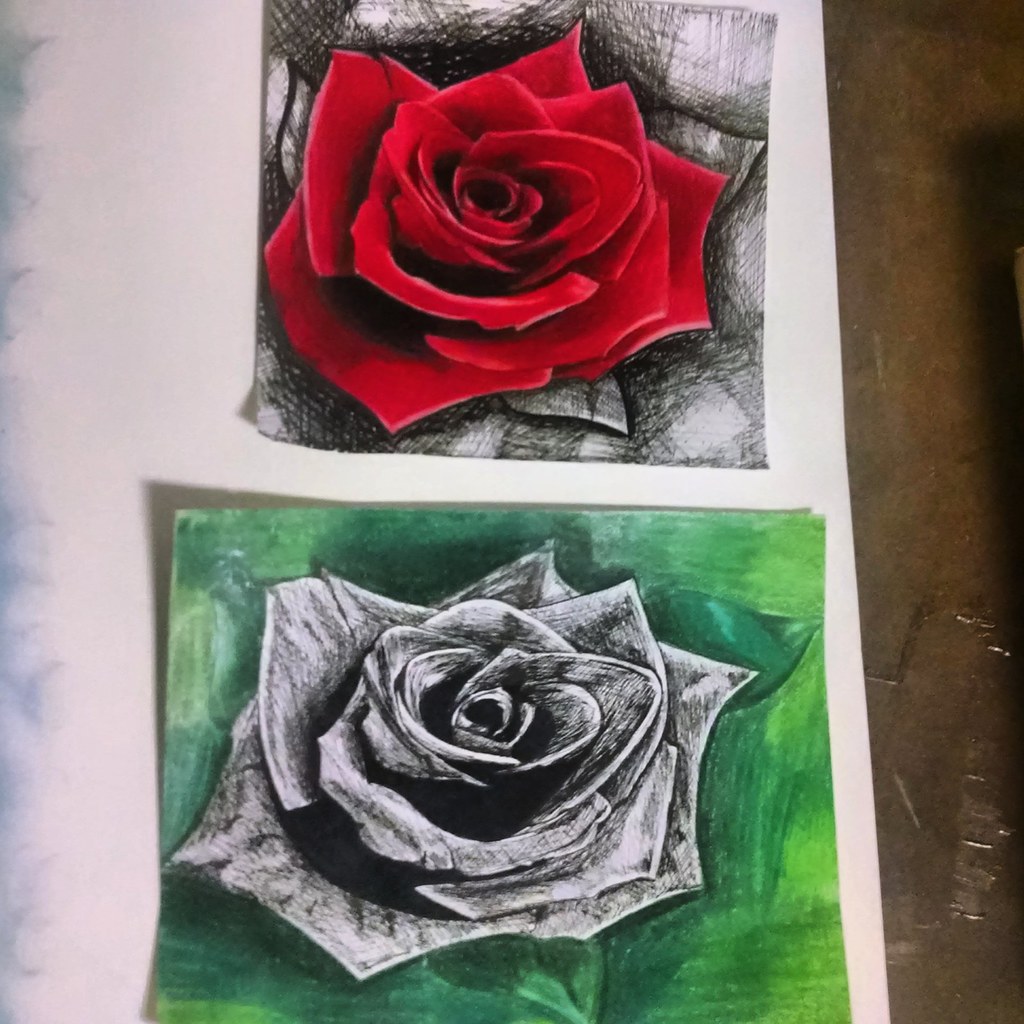The image showcases two intricate drawings of roses, each with distinct characteristics and backdrops. The top drawing features a vibrant red rose, meticulously shaded with black to enhance its depth. This rose is set against a striking black background that is accentuated by three additional white roses, providing a stark and elegant contrast. Below, the second drawing portrays a white rose, artistically shaded with black to create a monochrome effect. This rose is framed by a lush green background, complemented by two green leaves.

Both drawings are placed on a larger white poster board, which has a hint of blue shading on the left side, adding a subtle touch of color. This poster board rests on a brown table, where the bottom right corner reveals either broken glass or clear tape, adding an element of mystery and texture to the scene.